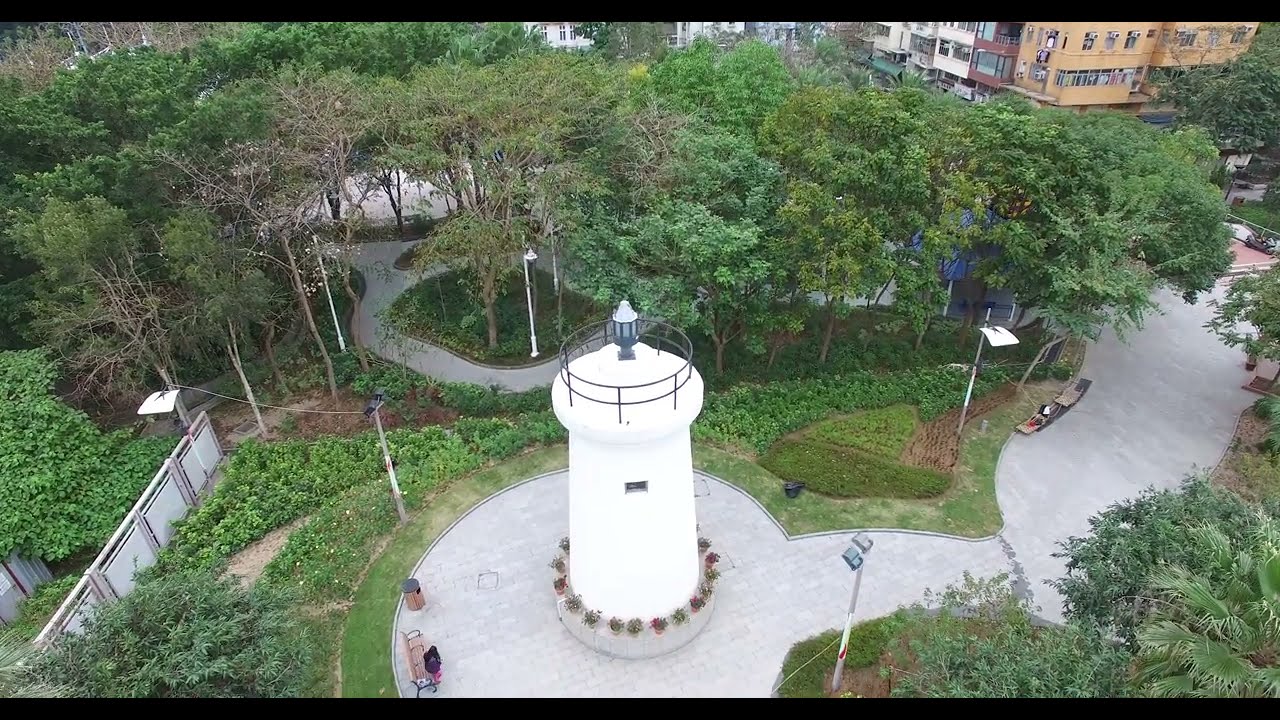This image is a detailed bird's-eye view of an athletic complex, prominently featuring tennis courts and an array of sports facilities. At the center lie two tennis courts with characteristic reddish floors bordered by tall blue metal fencing. The courts are easily identifiable by the green and blue interior markings typical of tennis. Surrounding these courts are rows of trees that appear to be evergreens, lending a natural backdrop to the scene.

In the foreground, resting on concrete pads, are green and blue long rowing boats, overturned atop sawhorses. These kayak-like vessels are neatly arranged, hinting at their use for competitive rowing activities. Interspersed around the background, there are a number of white, green, and yellow crates, seemingly scattered in an orderly fashion.

On the left and far back of the image, additional athletic facilities are visible, including a court that may serve either basketball or tennis, encircled by the same blue fencing. To the right, there's a larger field, likely used for soccer or field hockey, distinguished by its green turf and surrounded by a red rectangular track, all enclosed by blue fencing.

Overall, the complex is interconnected by concrete paths, and surrounded by greenery, with various trees and bushes enhancing the visual appeal. The entire layout appears well-organized, suitable for a variety of sporting activities, while also maintaining an orderly aesthetic.